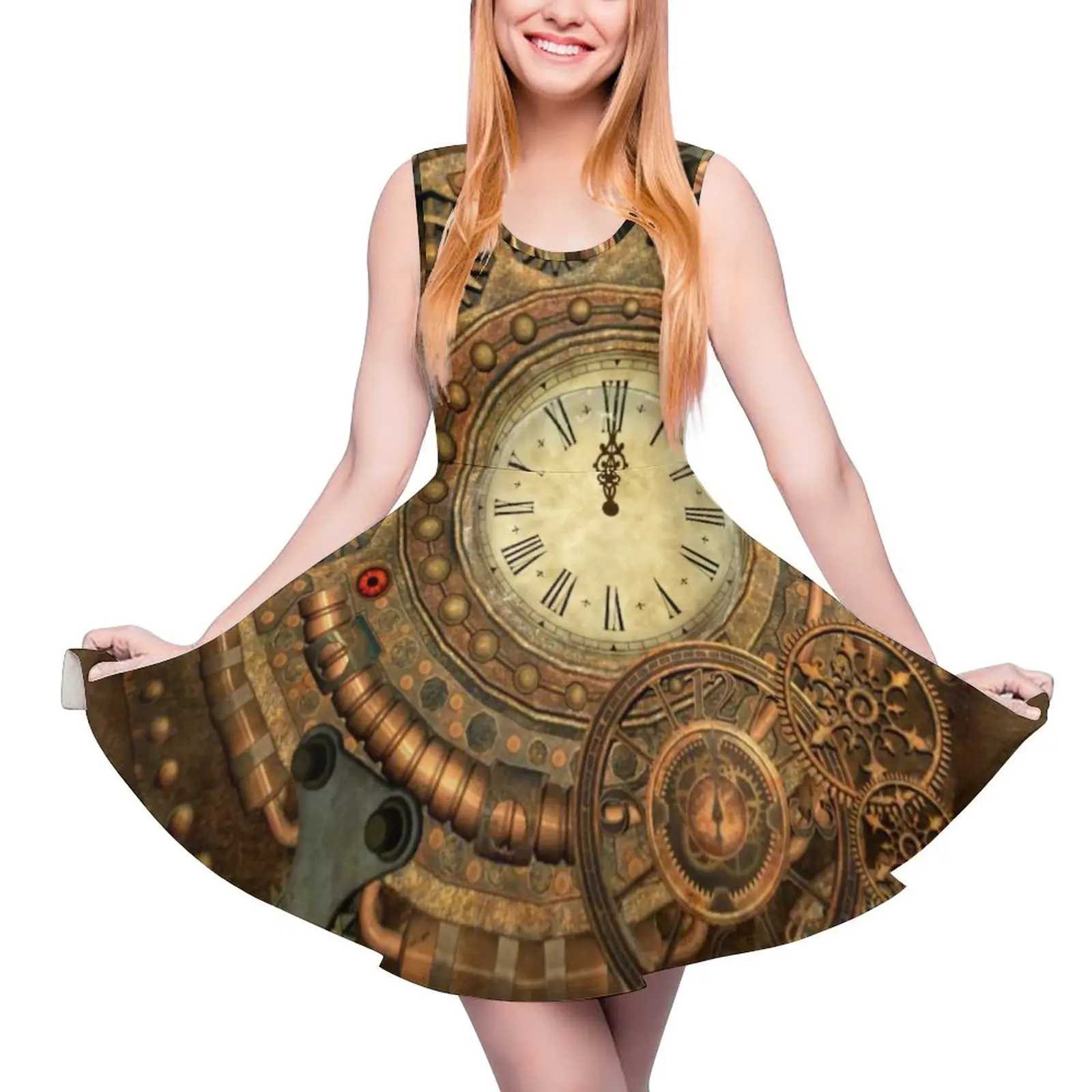The image showcases a product advertisement with a young woman in a fashionable, futuristic, steampunk-inspired dress. The woman's head is cropped off just above the nose, and the image cuts off just above her knees. She has pale skin, long blonde hair, and is smiling while holding her dress out with both hands, in a curtsy-like pose. The dress features a sleeveless design with a large, open neckline and short skirt. Its primary coloration is brown, adorned with an off-center clock face positioned by her waist. This clock face, set at 12 o'clock, is surrounded by intricate, photoshopped images of gears, copper, and brass elements, giving it a distinct Jules Verne or steampunk aesthetic. The background is entirely white, emphasizing the artistic and mechanical elements on the dress. The woman also appears to be wearing sheer tights and her entire arms and partially her legs are visible.